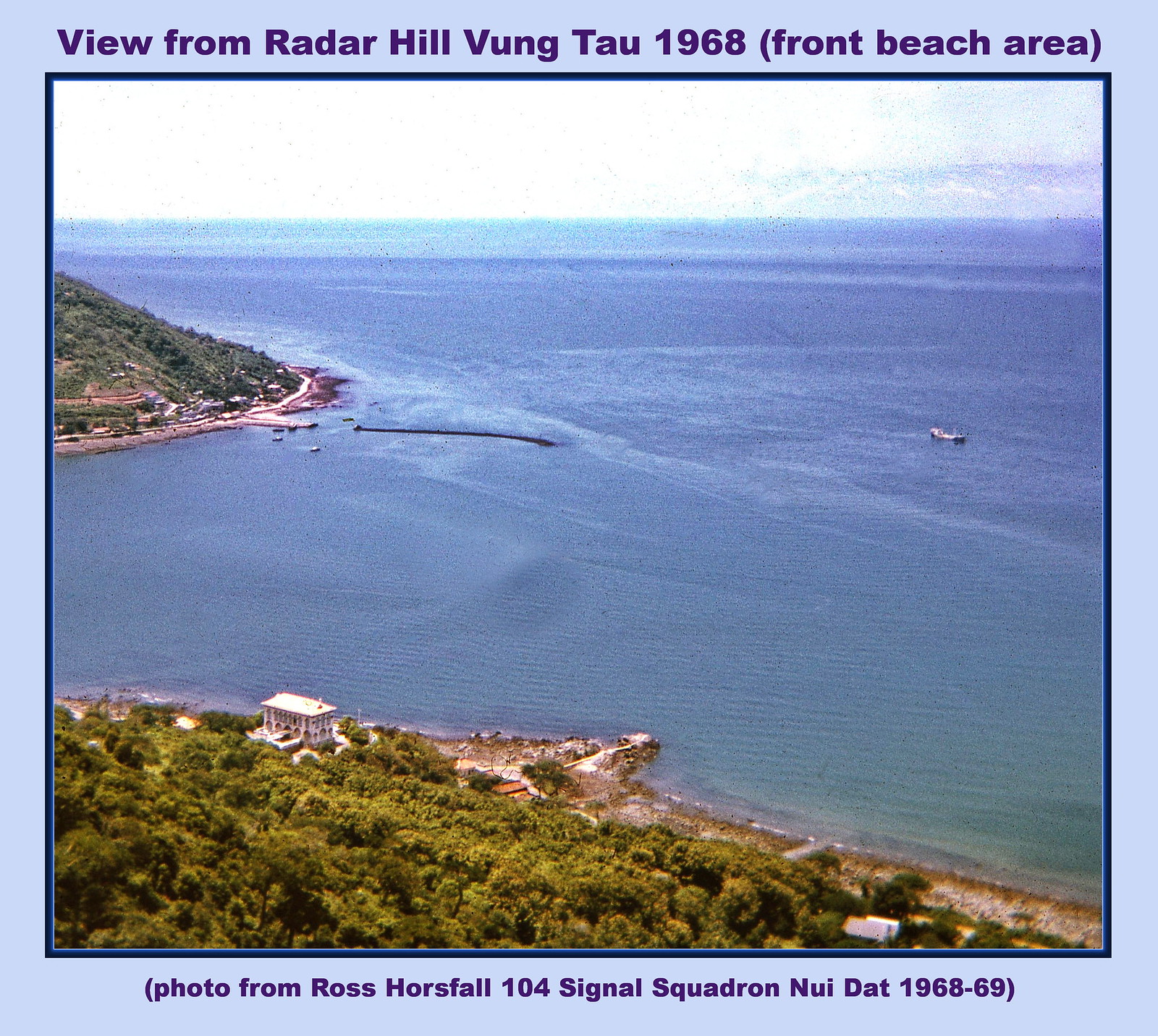The image captures a postcard-style view from Radar Hill, Vung Tau, 1968, prominently displaying the front beach area. At the bottom, it is noted as a photo from Ross Horsfall, 104 Signal Squadron, NUI DAT, 1968-1969. The scene is a coastal landscape featuring a vibrant mix of dark blue and turquoise waters, with visible sand dunes beneath the waves. Several white boats are scattered in the expansive blue water, with one moored near a docking station. On the coastline, rocky shorelines and a couple of hills are seen, one with a black structure jutting into the sea. There are white buildings, including a prominent house on the beach, with more buildings spread along the coast. The area is rich with rocky terrain, leafy trees, and grassy slopes, indicating a sunny day despite the sky appearing a bit whited out. Lastly, a blue line outlines the entire picture, and purple text above and below adds a historical and personal touch to the image.